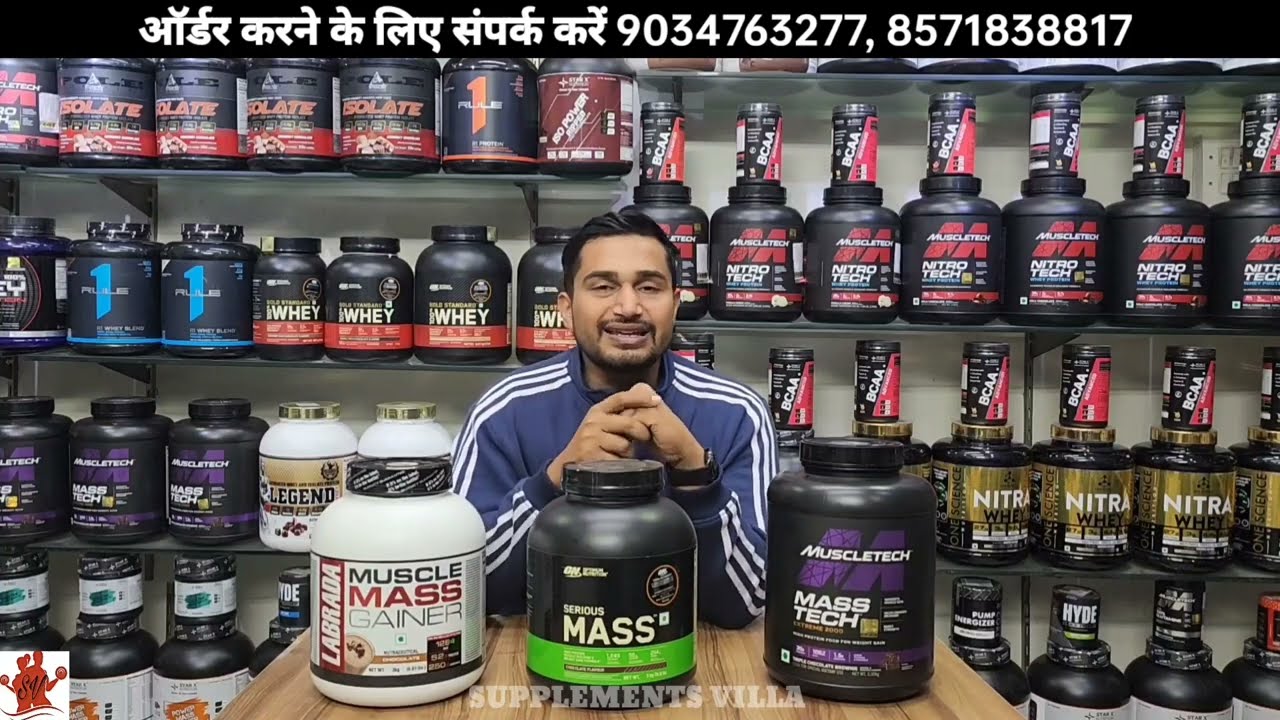In this image, we see an advertisement set in what appears to be a supplement store, featuring a man, possibly of Indian or Middle Eastern descent, promoting various muscle mass-gaining products. At the top of the image, there's a thin black header with white text in a foreign language, potentially Indian, alongside two phone numbers: 903-476-3277 and 857-183-8817. The man, who has brown skin, short straight black hair, and a closely trimmed black mustache and beard, is standing behind a wooden table, smiling directly at the camera. He is wearing a blue jacket with white pinstripes. 

On the table in front of him are three large containers of muscle gain supplements. The one on the left is white and is labeled "Muscle Mass Gainer by Labrada". The middle one is black with a green banner labeled "Serious Mass". The one on the right is also black and is labeled "Muscle Tech, Mass Tech" with a purple logo behind it. There is also text towards the bottom of the image that reads "Supplements Villa," which is semi-transparent. 

In the background, several shelving units are loaded with numerous containers of similar muscle gain and workout powders. The colors in the image are predominantly black, gray, blue, red, orange, gold, and purple. In the lower right corner, a red silhouette logo of a man and woman lifting weights is visible, further emphasizing the fitness theme of the store.